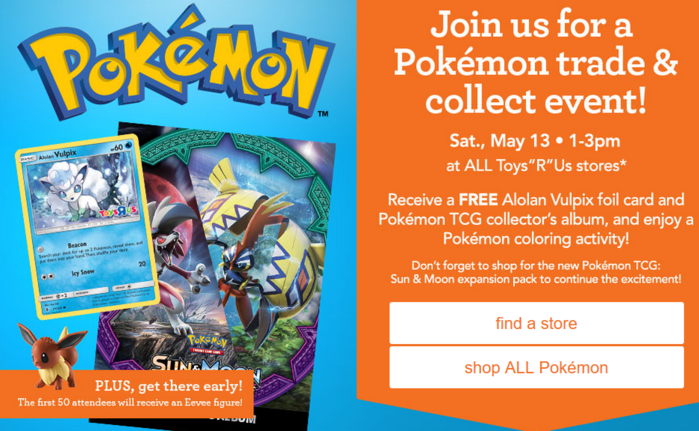**Join the Excitement!**

On the left side of the advertisement, the backdrop is a vibrant blue with bold yellow-orange text at the top proclaiming "Pokemon," each letter outlined in blue. Below this header, an image of a Pokemon card featuring Vulpix is shown, although the text is somewhat blurry. The Vulpix, depicted as an animal with a thick white mane and four hooved legs, takes center stage on this card. Beneath the Vulpix card, another image showcases Pokemon characters with the text "Sun and Moon" prominently displayed. Adjacent to this is a picture of a brown, long-eared Pokemon, accompanied by the message: "Plus, get there early. The first 50 attendees will receive an Eevee figure."

To the right side, the background shifts to a bright orange with crisp white text that reads: "Join us for a Pokemon trade and collect event. Saturday, May 13, 1-3 PM at all Toys R Us stores." It further details the perks: attendees will receive a free Alolan Vulpix foil card and a Pokemon TCG collector's album, in addition to enjoying a Pokemon coloring activity. The invitation encourages attendees to "shop for the new Pokemon TCG Sun and Moon expansion pack to continue the excitement."

Below this section, a white triangle with orange text urges viewers to "Find a store," and an adjacent white rectangle with centered orange text prompts them to "Shop all Pokemon."